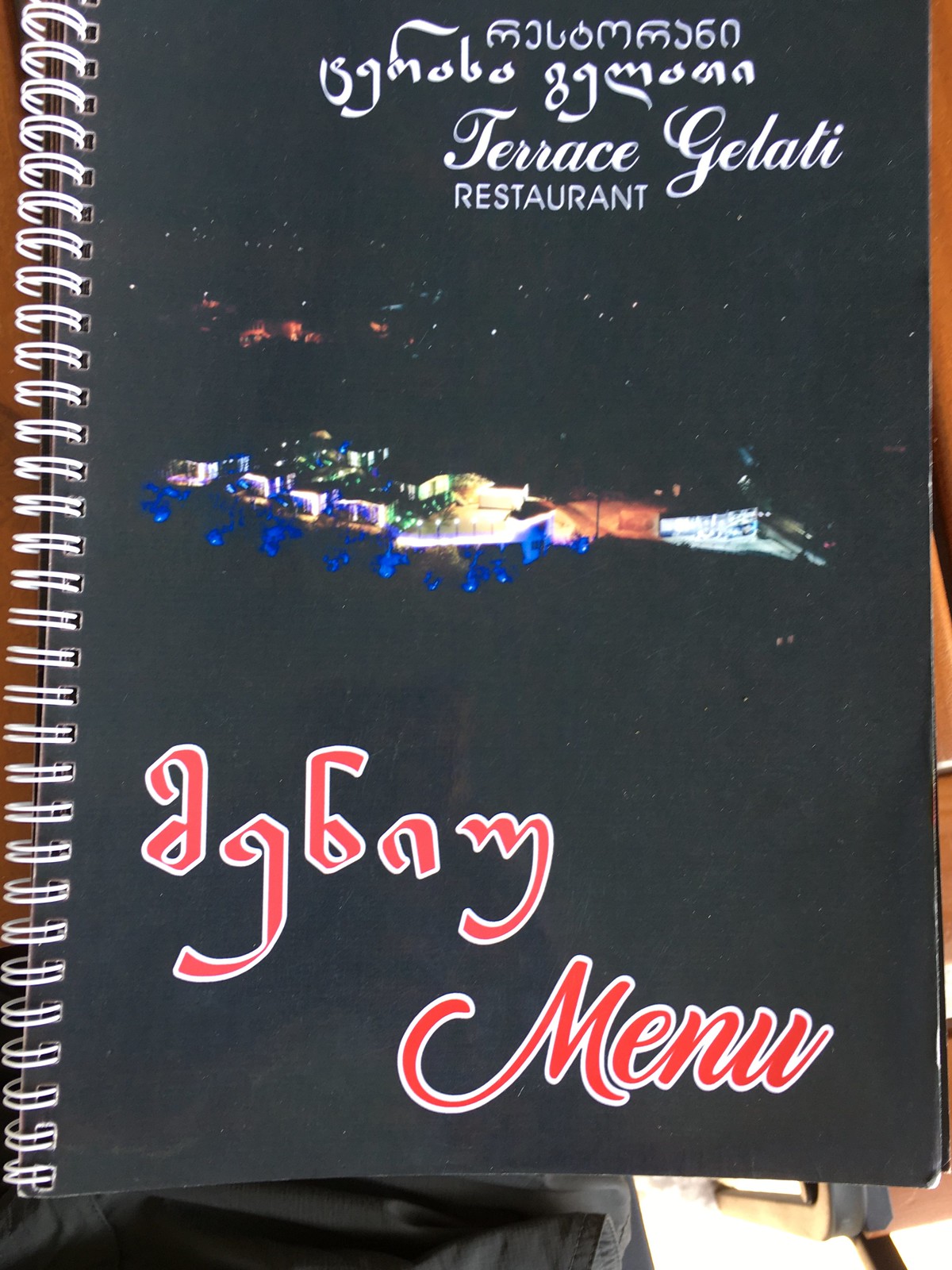A spiral notebook, serving as a menu for "Terrace Gelati Restaurant," is depicted. The cover features the restaurant's name prominently at the top in white text, alongside some phrases in a different language. The word "Menu" is written at the bottom in red, outlined in white. The background of the cover is predominantly black, providing a striking contrast to the text and other design elements. The notebook is bound with a double white spiral. Centrally, there is a dark, nighttime aerial photo of the restaurant, likely taken from a drone or aircraft. The image shows the restaurant illuminated, with blue lights accentuating the building and its surroundings, giving an enchanting and inviting look.